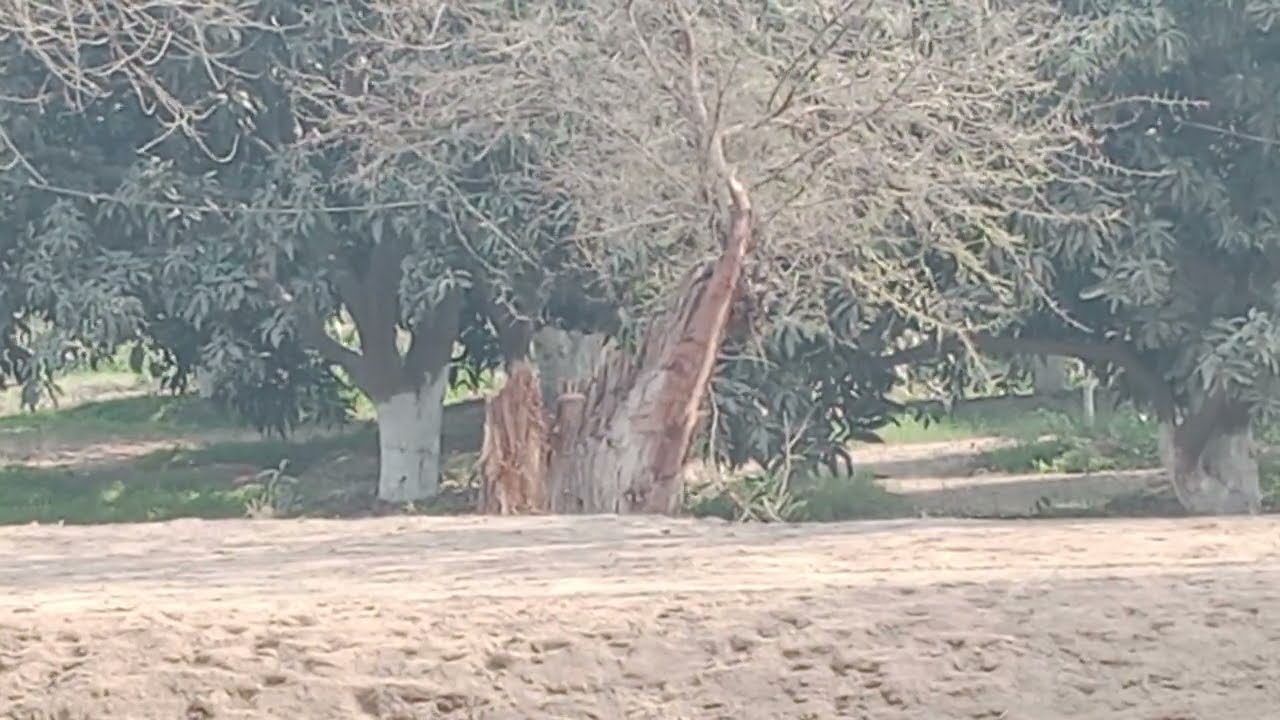This daytime photograph captures a natural scene in what appears to be a park or beach setting. In the foreground, there's a large expanse of pale, beige sand with numerous footprints and indentations, suggesting the presence of people or animals. The sand transitions into trails that weave through the scene, bordered by patches of green grass.

The focal point of the image is a prominent tree in the center. This tree stands out due to its very light, almost white-colored branches, indicative of possible ill health. Its trunk has a beige, almost orange tint and appears partially snapped, with an absence of leaves despite the abundance of branches resembling nerve endings. 

To the left and right of this central tree are more traditional-looking trees. These feature brown trunks with white-painted bases and are covered with lush, green leaves, contrasting starkly with the central tree. Together, these elements create a rich, detailed portrayal of a natural landscape, capturing both the serene and intricate aspects of the scene.